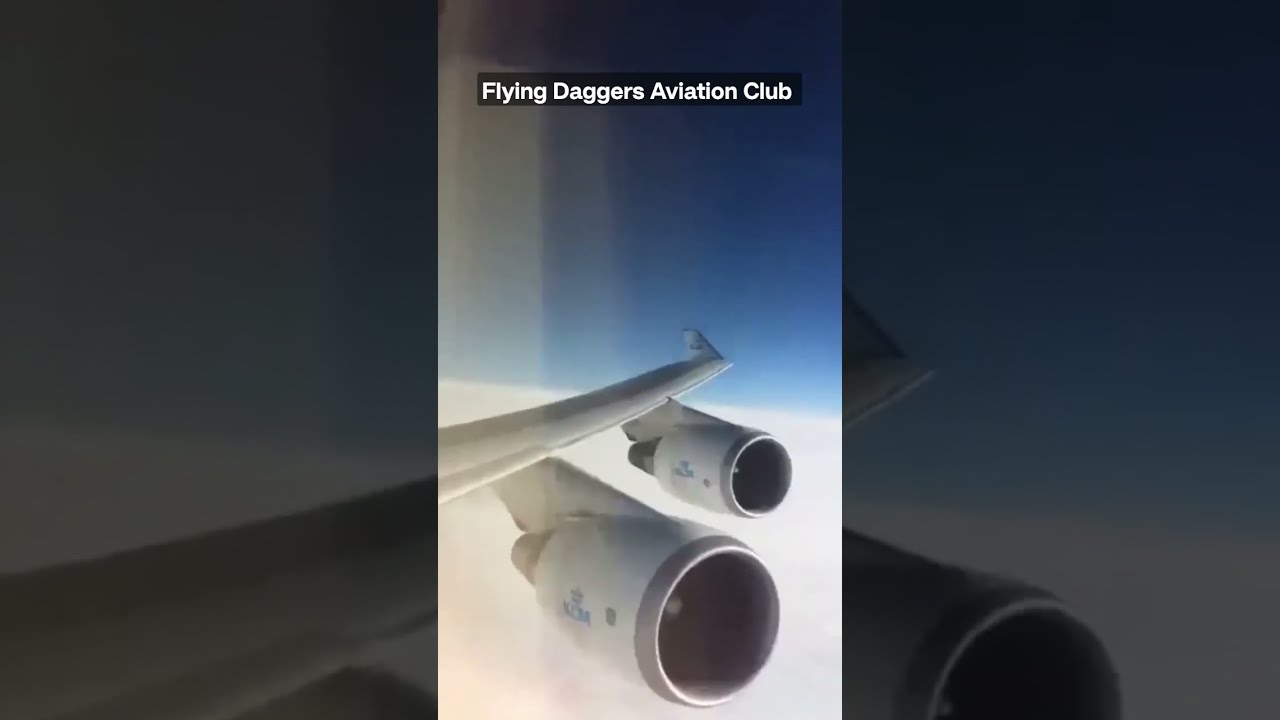The image is a horizontal rectangle featuring a photograph of an airplane wing with two cylindrical white jet engines, viewed from an airplane window. The engines have gray circular borders around their outer edges, and they're mounted on a big silver wing. The view overlooks a thick blanket of white clouds below, with a light blue, starless sky above. The image is somewhat blurry and hazy but captures the essence of being high up in the air. At the top of the image, on a black horizontal bar, is the text "Flying Daggers Aviation Club" in white letters. The background of the image mirrors the central photograph, creating a cohesive, albeit blurry and dark, frame around the main picture.